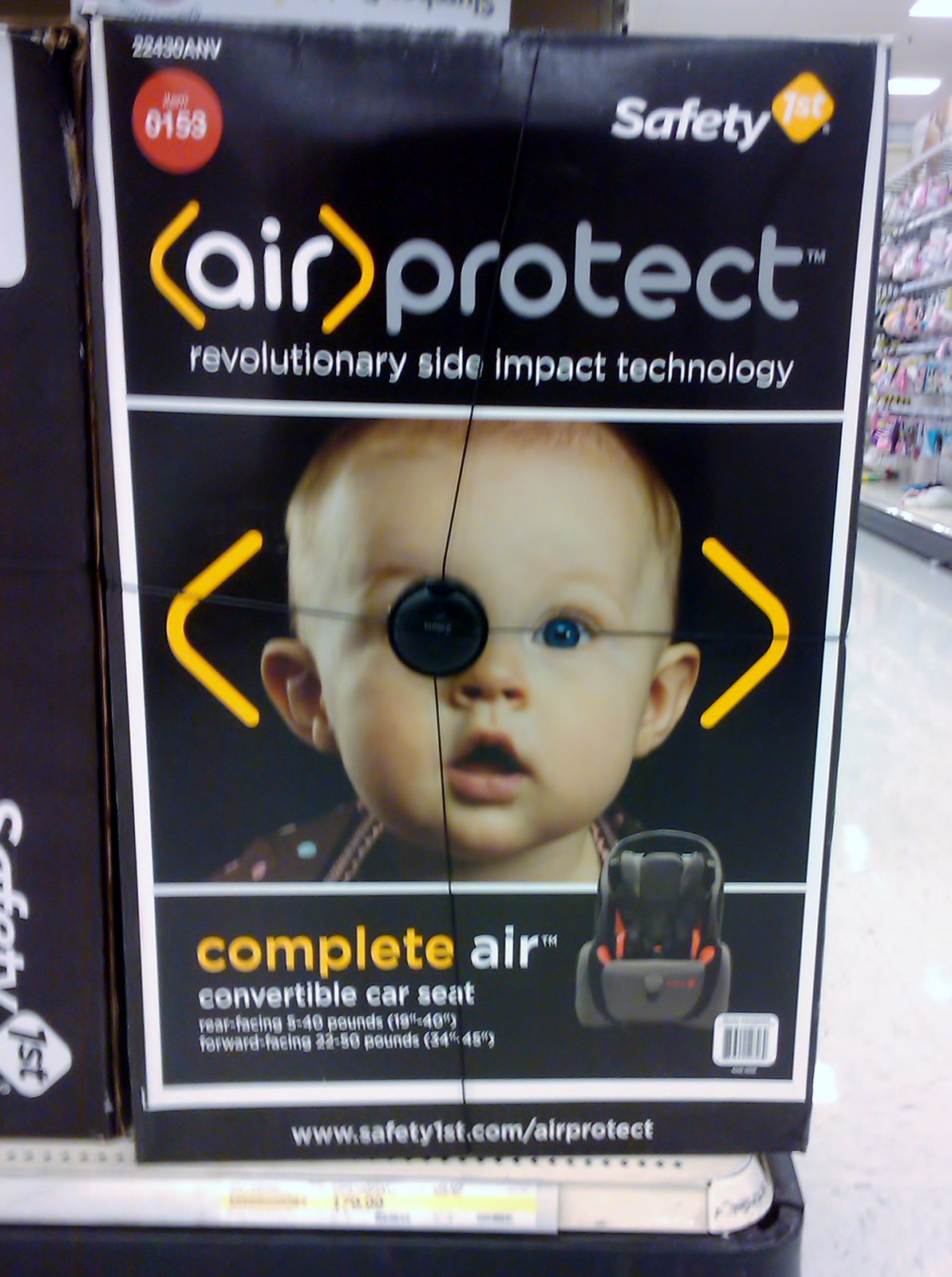The image captures a boxed baby's car seat taken in an indoor store setting, prominently displayed on a shelf with a price tag beneath it. The mostly black box features a large photo of a cute baby with blue eyes and wearing a brown shirt with blue polka dots, positioned at the center. Notably, a black anti-theft tag covers one eye, giving the baby an eye-patch appearance. In the top right corner, "Safety 1st" is displayed in white lettering within a yellow diamond. Below this, the box proclaims "Air Protect" in yellow parentheses, followed by "Revolutionary Side Impact Technology."

Underneath the baby’s image, "Complete Air" is written, with "Complete" in yellow and "Air" in white text. There is also a small visual of the car seat in black and orange at the bottom right, tagged as a convertible car seat. The descriptions include "Rear-Facing: 5 to 40 pounds, 19 to 40 inches" and "Forward-Facing: 22 to 50 pounds, 34 to 45 inches." The bottom of the box directs viewers to "www.safety1st.com/airprotect." To the right of the primary display, other baby merchandise hangs on fixtures across the aisle.